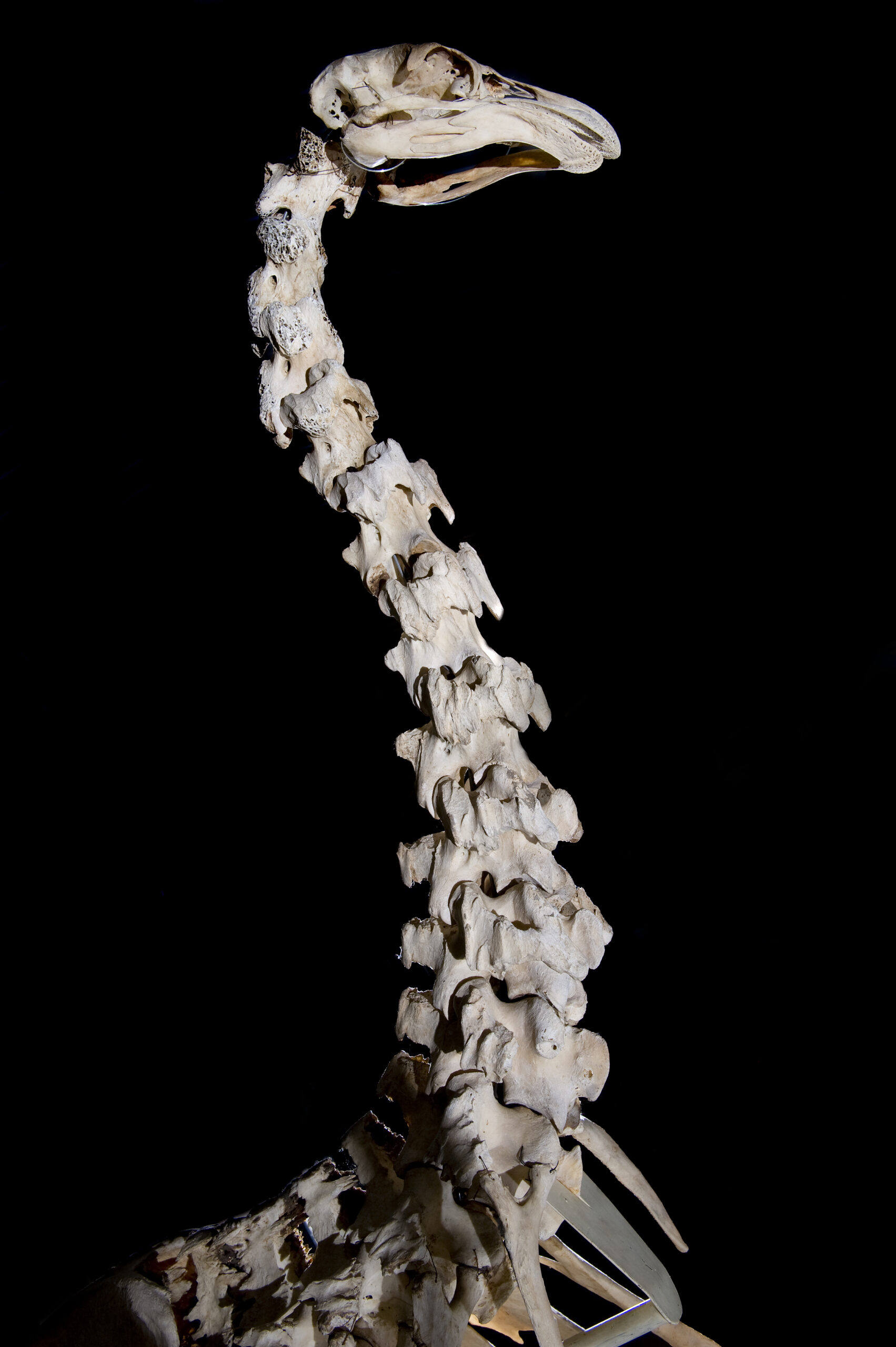This image depicts the skeletal remains of a long-necked creature, possibly a prehistoric bird, swan, or even a giraffe, set against a stark black background with bright, focused lighting. The neck, elongated and slightly S-curved, features a clearly defined spinal column with numerous vertebrae. At the top of the spine is a small, thin skull adorned with a beak, hinting at a bird-like origin. The bottom of the spine extends downwards but is abruptly truncated, leaving much of the lower body obscured. Emerging from the lower spinal area are structures resembling short appendages or spikes, which add to the complexity of the skeletal display. The bones, creamy and faded in color, exhibit some spongy textures and are supported with pins and wires that secure the ribs and potential forelimb structures. A metallic object, possibly a disc, is visible within the skull, likely serving as reinforcement for the skeleton's display. This striking composition is both scientifically intriguing and visually captivating.